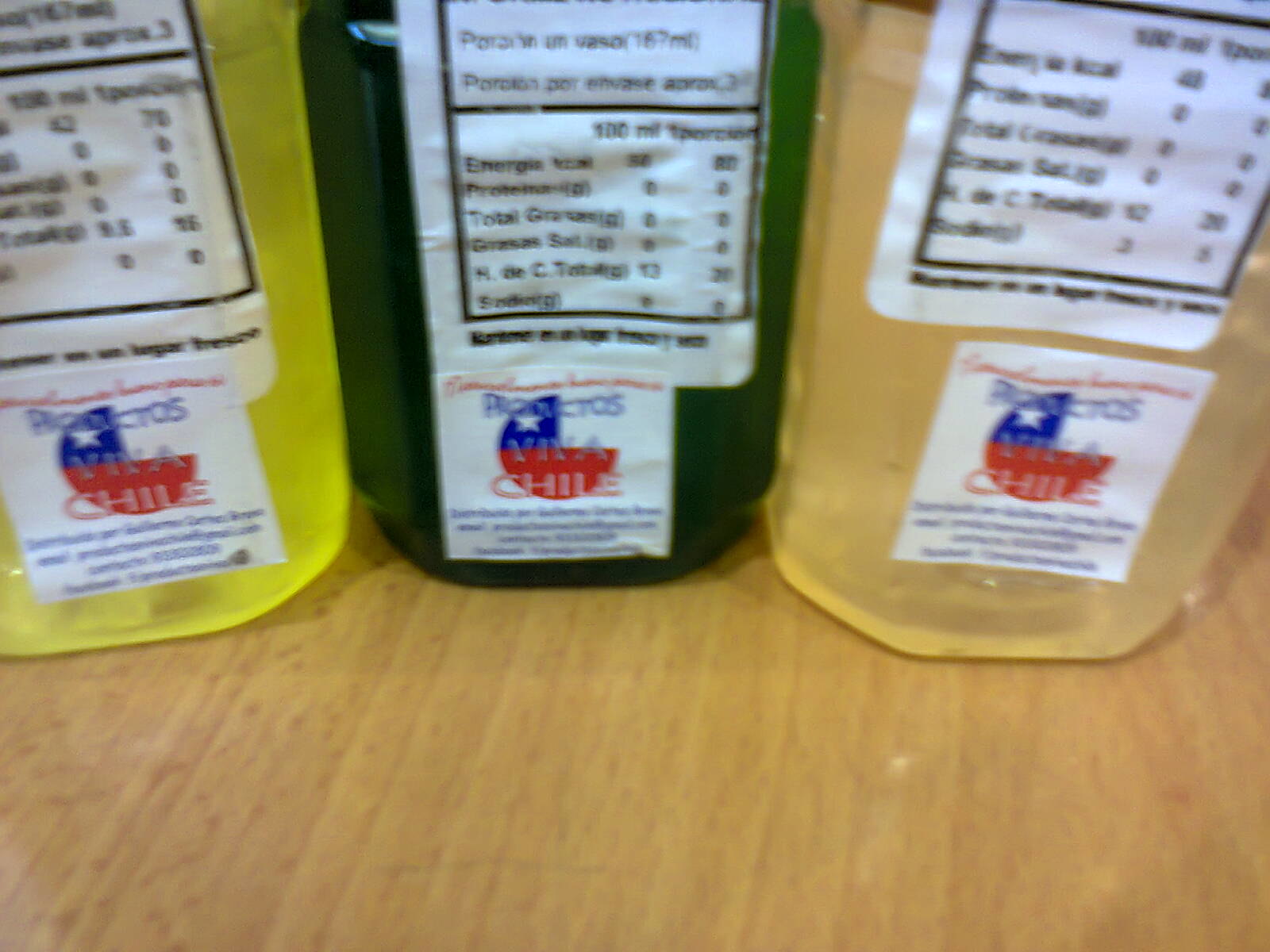The image showcases a close-up shot of a light-colored, golden brown tabletop, likely a formica surface mimicking wood. Resting on it are three distinct plastic containers, each with slightly blurry details. The container on the left is a bright yellow and resembles a lemonade-like bottle. The middle container is green, and the right container is a pale beige, potentially hinting at apple juice. Each container prominently displays a nutrition facts label, though the text is unreadable. Beneath these labels, there are square white stickers, each bearing a red, white, and blue symbol with a white star, alongside the words "Productos Viva Chile." The presence of Spanish text on the labels indicates they likely contain consumable or food products, with the word "chili" being the only legible term.